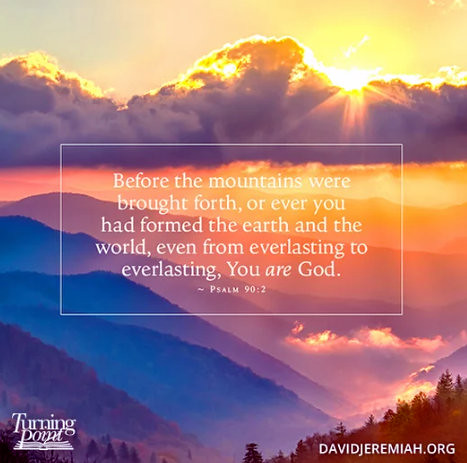The image is a square-format card featuring a beautifully filtered photograph of a mountainous landscape during sunset. The background showcases a gradient of colors from yellow, orange, and purples to blues and browns, with hazy mountains and dark green trees in the foreground. A dark gray cloud partially conceals the sun, creating a serene sky with a vivid color gradient effect. Superimposed in the center is a white rectangular outline, containing an inspiring Bible verse in white typography: "Before the mountains were brought forth, or ever you had formed the earth and the world, even from everlasting to everlasting, you are God. Psalm 90:2." The bottom left corner holds an underlined "Turning Point" logo, and the bottom right corner displays "DavidJeremiah.org" in white text.